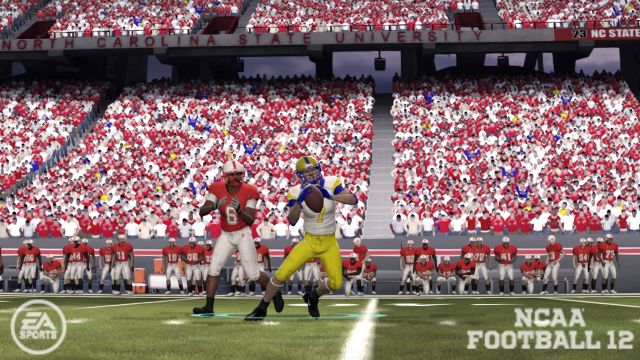This screenshot is from the video game "NCAA Football 12," as indicated by the white font in the bottom right corner. On the left side of the screen, the EA Sports logo is prominently displayed within a circular icon. The scene depicts a college football game taking place at North Carolina State University, evidenced by the university's name emblazoned in the stands. The stadium is filled with fans dressed predominantly in red and white to support the home team. The action on the field features two players: one donning a red and white uniform, and another in blue, gold, and white, who is seen holding a football while running across the green field adorned with white lettering.